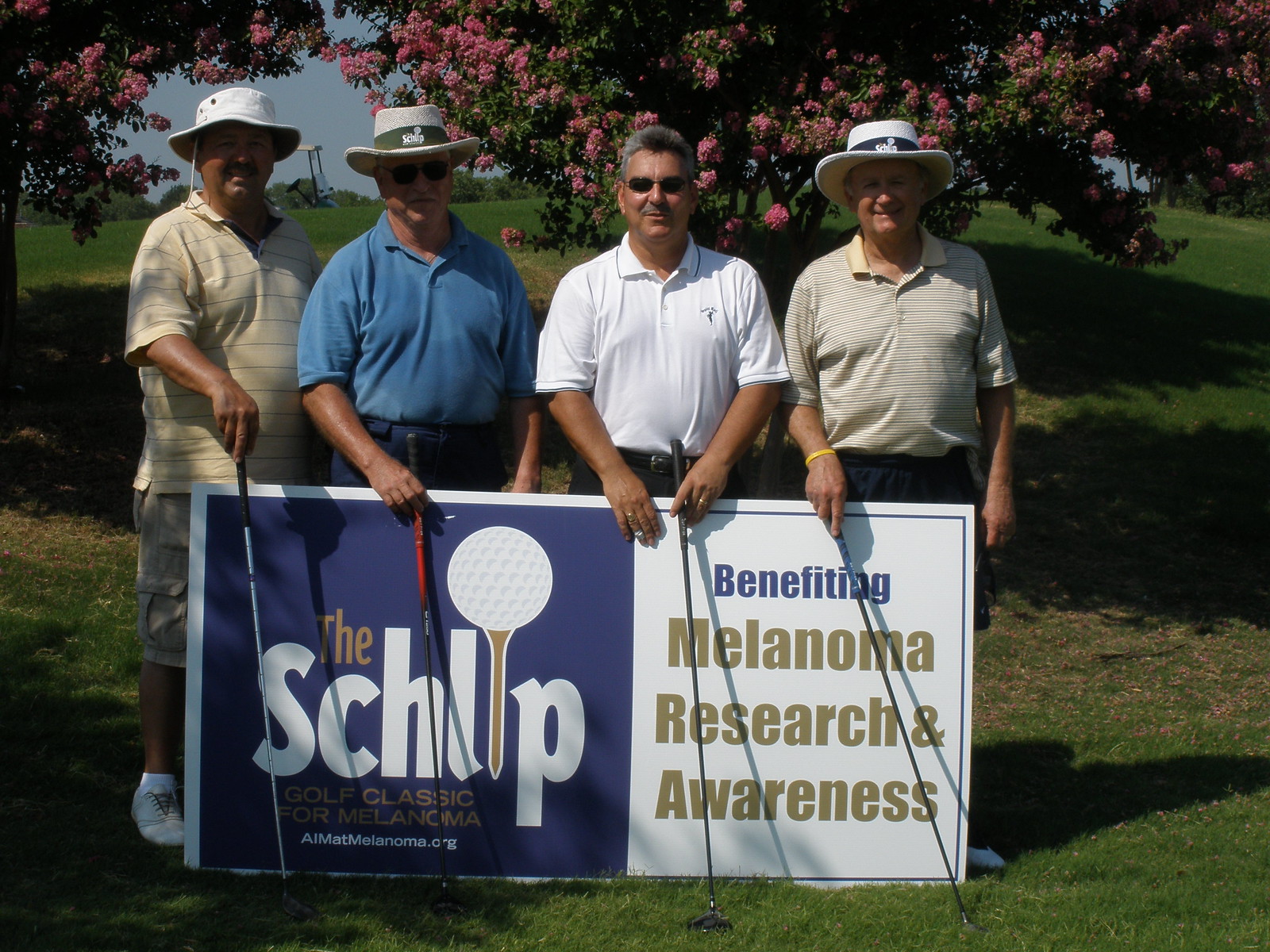The photograph captures an outdoor setting with four men standing in a straight line, holding golf clubs in front of a banner. The banner prominently reads "The Schlip" with the 'I' stylized as a golf tee with a golf ball. Below this, the text reads "Golf Classic for Melanoma," and further down, "Benefiting Melanoma Research and Awareness" is displayed along with a URL. From left to right, the man on the left wears shorts and a beige striped shirt, complemented by a white sun hat. Next to him, the man in a blue shirt with blue pants sports a white hat with a green band and sunglasses. The third man is in a white shirt with black pants and wears sunglasses. The man on the far right wears a striped, beige shirt, dark shorts, and a hat. Behind them, the lush greenery of a golf course is visible, including a gnarled tree blossoming with pink flowers and a parked golf cart to the left. The image effectively highlights their commitment to melanoma research and awareness.